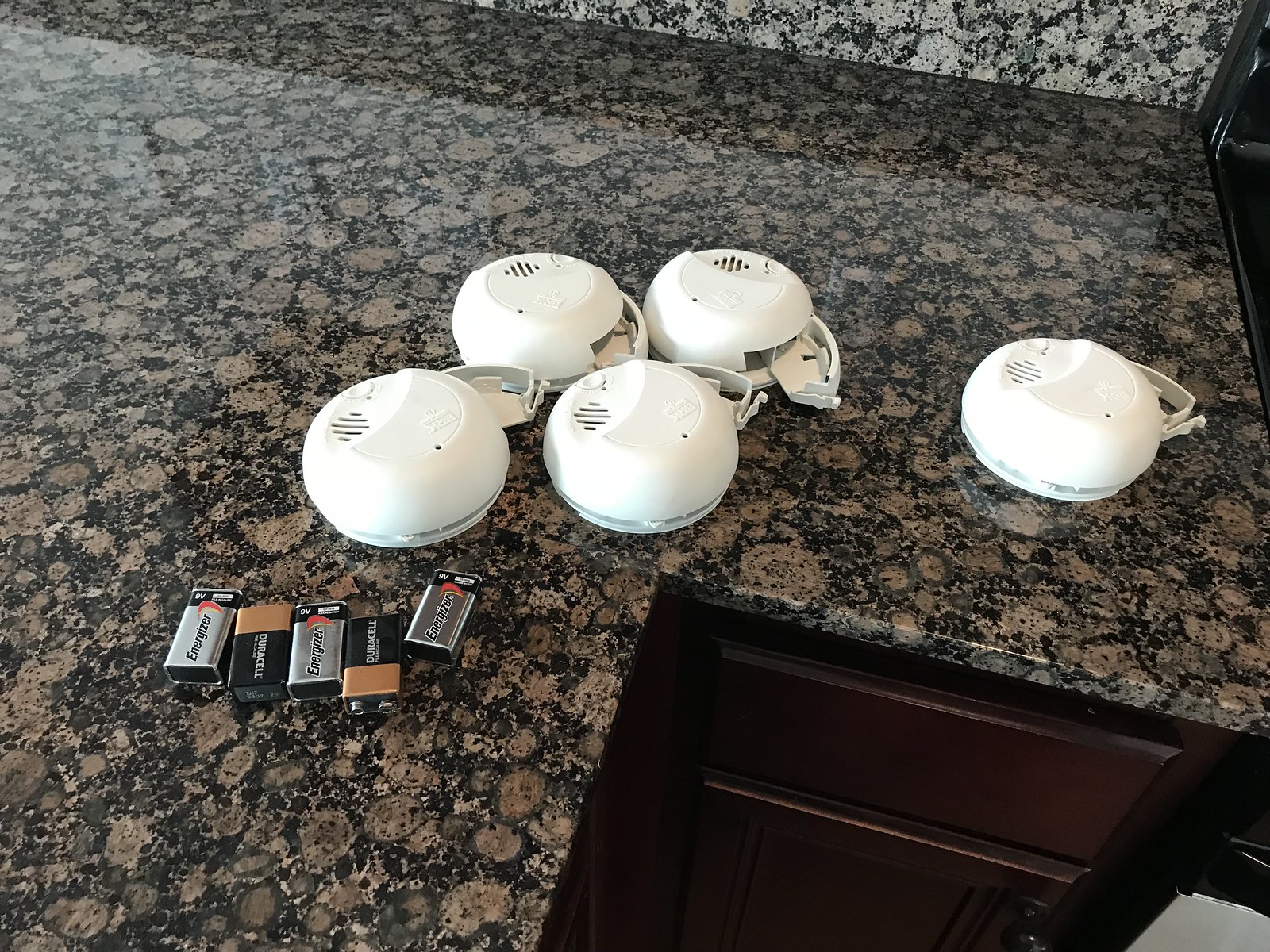The image depicts a collection of five white smoke detectors arranged on a glossy, dark granite countertop with purple and lighter gray splotches. The countertop, likely part of a kitchen setup, is positioned at a slight angle, revealing dark brown cabinetry below. All five smoke detectors have their battery compartments open and empty, facing the right. In the foreground, five 9-volt batteries are laid flat on the countertop, neatly lined up with a mixture of three Energizer (silver and black) and two Duracell (gold and black) batteries. One smoke detector stands slightly apart from the cluster of four in the center. The countertop's reflective finish juxtaposed with the simple, white design of the smoke detectors creates a clean, organized scene.